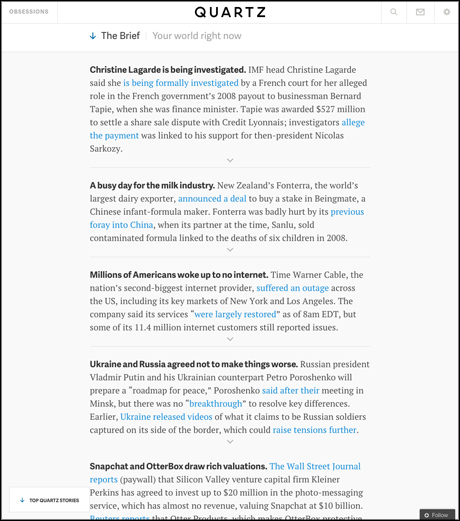Set against a clean white background bordered by a precise black line, the image captures a screenshot of a web page. In the upper left corner, there is the section header labeled "Obsessions" rendered in subtle gray text. Centrally positioned at the top of the page, the bold black text "Quartz" identifies the website. The upper right corner hosts three familiar icons in grayscale: a magnifying glass for search, an envelope for mail, and a cogwheel for settings.

Beneath these header elements, a prominent white banner spans across the page, carrying the message "Your World Right Now" alongside a brief descriptor, "The Brief," accompanied by a downward-pointing blue arrow indicating more content below. 

The main content highlights breaking news headlines. The foremost headline, "Christine Lagarde is being investigated," reports that the IMF head, Christine Lagarde, has announced she is under formal investigation. The phrase "is being formally investigated" serves as a clickable link, likely leading to the full article.

Directly beneath this, another headline in bold black text reads, "A Busy Day for the Milk Industry," hinting at significant developments or events within the dairy sector. The final headline in view states, "Millions of Americans Woke Up to No Internet," signaling widespread internet outages affecting a massive number of people.

This composition succinctly captures the key elements and current headlines of the Quartz web page within a neatly framed screenshot.